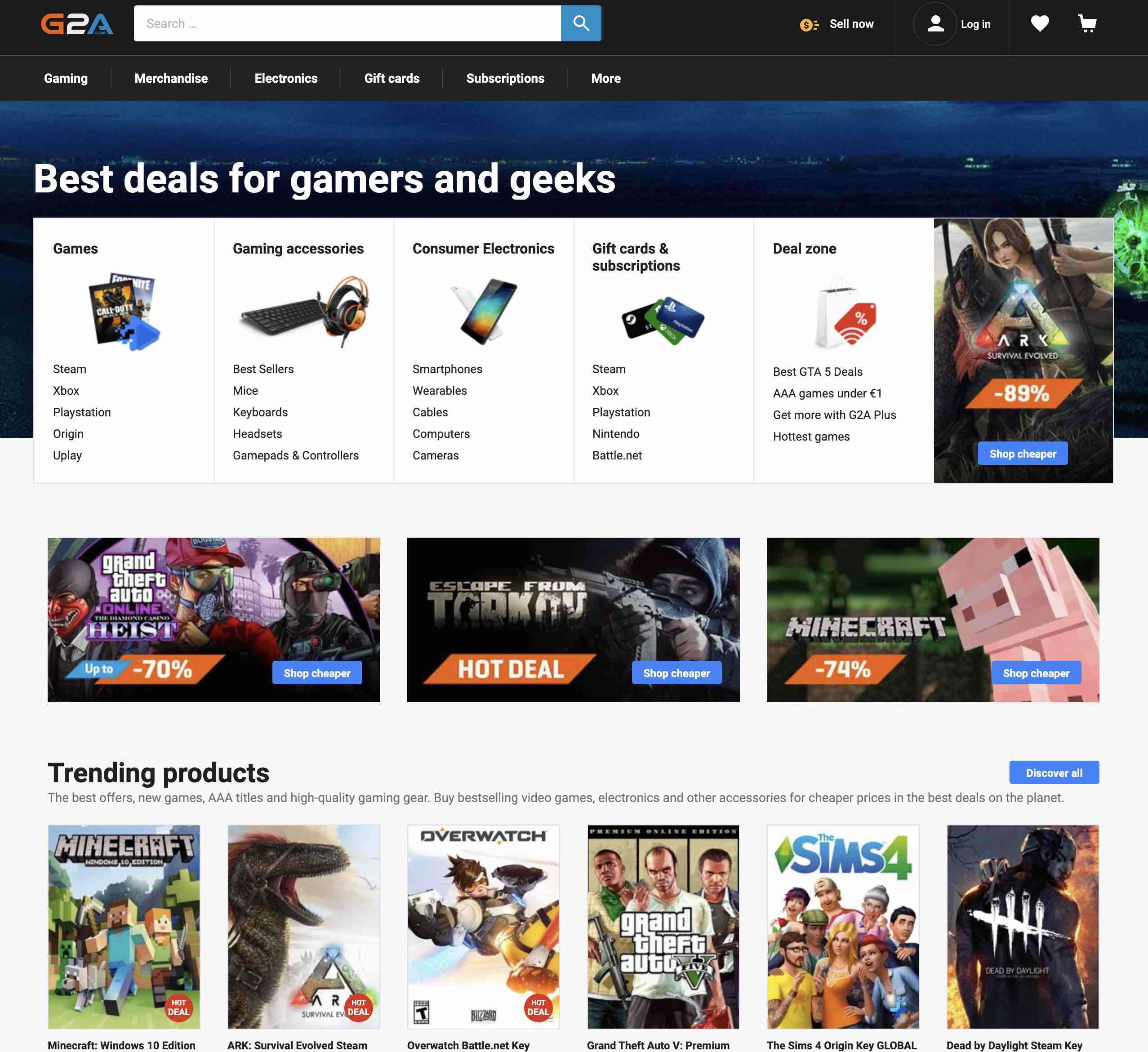The image is a screenshot of a web page for a gaming retail platform, identified by the logo "G2A" written in red, white, and blue, situated in the top left corner. To the right of the logo, there's a functional search bar. Further right, the top navigation includes icons and links for "Sale Now," "Login," a heart (presumably for a wishlist or favorites), and a shopping cart.

Just below this navigation bar, there is a secondary menu offering detailed categories such as gaming merchandise, electronics, gift cards, and subscriptions. 

Prominently featured beneath this menu, the page boasts a headline in white text on a dark blue background that says, "Best Deals for Gamers and Geeks." 

Following the headline, there are multiple categorized sections each coupled with product images. The categories include games, gaming accessories, consumer electronics, gift cards and subscriptions, and the "Deal Zone."

Highlighted are specific game deals with accompanying artwork, featuring notable titles such as "Grand Theft Auto Online," "Escape from Tarkov" (correcting the previously misheard name "Torquay"), and "Minecraft."